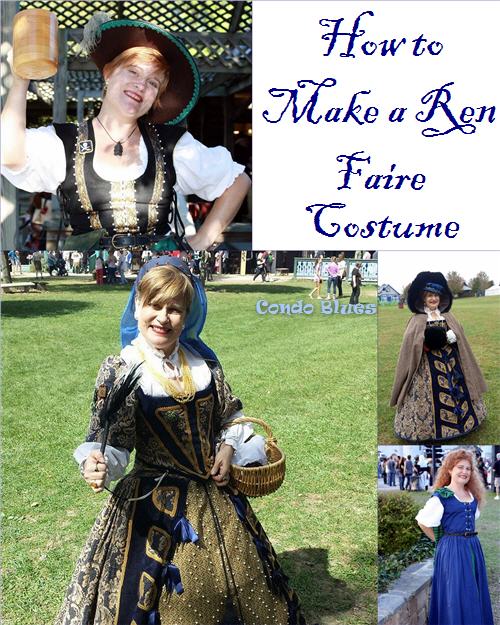The image is a promotional collage for an article titled "How to Make a Ren Faire Costume." The title is prominently displayed at the top right in a white square with blue text. The collage features four photographs showcasing different Renaissance fair costumes. 

In the top left photograph, a woman is shown from the waist up, dressed in a black vest with gold suspenders over a white short-sleeve blouse. She wears a brown hat with a green rim and holds a large wooden beer stein in her hand. Below this image, another woman is pictured from the ankles up, wearing an elaborate blue and gold dress with a matching blue bonnet. To the right of these two images, two more women are shown in similar Renaissance-style outfits, each wearing unique costumes that reflect the vibrant colors of blue, green, gold, and red. The overall setting emphasizes the diverse and intricate designs suitable for a Ren Faire costume.